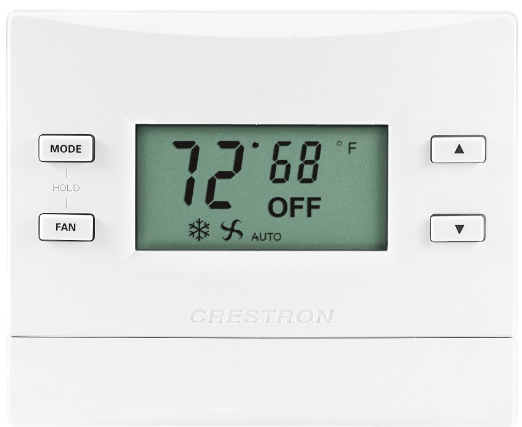The image showcases a white, square-shaped thermostat prominently displaying its brand, Crestron. The device appears to be a professional product image, possibly from the manufacturer's website, providing a clean, clear view of the device’s interface and design. 

At the center of the thermostat is a small digital screen. The largest text on the display reads "72 degrees Fahrenheit" on the left side, indicating the current room temperature. Adjacent to this, on the right, is a smaller display showing "68 degrees Fahrenheit" with the word "Off" positioned below it.

Two distinct symbols are visible on the screen: a snowflake and a fan with four blades, alongside the word "Auto," suggesting different operational modes for heating and cooling. To the left of the screen, there are three buttons labeled "Mode," "Hold," and "Fan" from top to bottom. On the right side of the screen, a pair of arrow buttons allow for temperature adjustments, with the upper arrow pointing upwards and the lower arrow pointing downwards.

Below the screen, the Crestron brand name is engraved directly on the device, exuding a sense of quality and craftsmanship. Additionally, there is a detachable panel beneath the branding, which possibly provides access for maintenance or additional controls, ensuring ease of use and functionality.